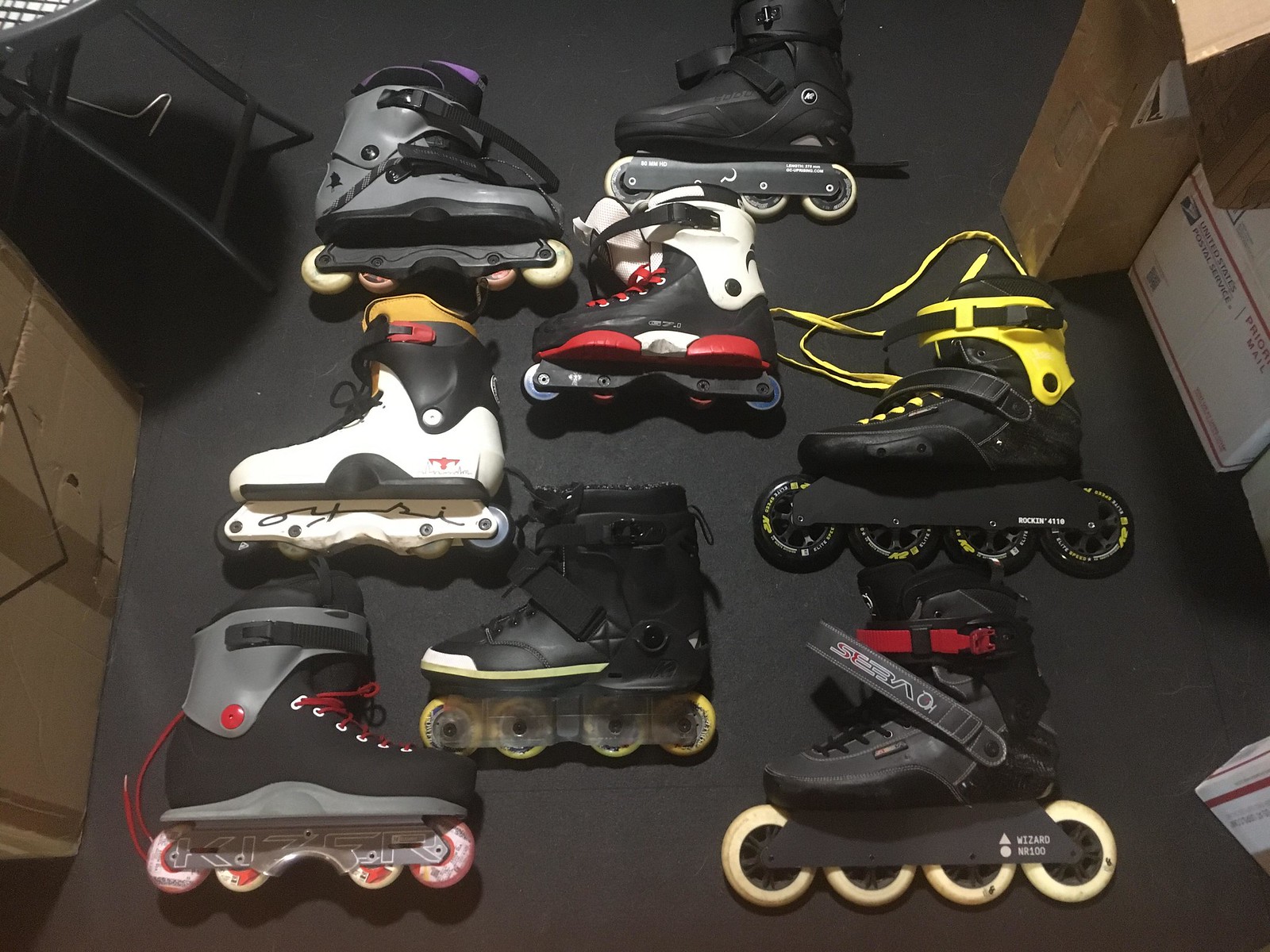The image depicts an aerial view of eight roller blades, arranged neatly on a black foam floor. The skates display a striking variety of colors and designs, each pair different from the others. From the top left, there is a gray skate with purple trim and dirty white wheels. Adjacent to it on the right is a black skate with white blades. Below it lies another black skate featuring a white lip and a hint of red on the sole. Midway on the left, there is a white skate with black text detailing on the white plastic near the blades. To the right, a black skate with conspicuous yellow laces and black wheels adorned with yellow text catches the eye. Further left, another black skate showcases a clear plastic blade holder with yellow blades. At the bottom left, a black and gray skate with red laces and some pink accents rests alongside white wheels. Lastly, the right-most skate is a plain black shoe. The background reveals additional details including cardboard boxes, one marked with a United States Postal Service Priority Mail label, and the legs of a table with a small hook underneath. Overall, the arrangement accentuates the variety and individuality of each skate, creating a visually engaging display.